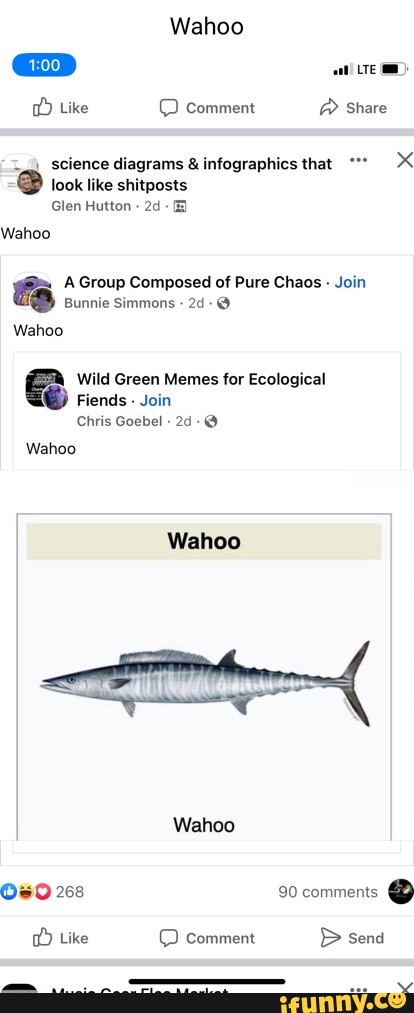A person is viewing their Facebook feed on their phone, with the screen prominently displaying several posts prominently featuring the word "Wahoo." The top part of the screen shows the Facebook header, while below is a series of posts shared by various users.

In the first post, Glenn Hutton shared content from a group known for its chaotic and humorous nature. The post originally shared by Bunny Simmons two days ago features the phrase "Wahoo" and falls under the theme of science diagrams and infographics that resemble humorous shitposts. 

The next post is shared by Chris Goble, also from two days ago, from a page named "Wild Green Memes for Ecological Friends." This post mirrors the phrase "Wahoo" and features an image of a long, slender fish. The fish depicted has distinct tiger-like stripes, a pointed mouth, a boomerang-shaped tail, and two fins situated in the middle of its body. Additionally, it sports a distinctive mohawk-like fin running down its back.

This particular post has garnered significant attention, receiving 268 reactions in total, including likes, funny face emojis, and hearts. It has also sparked considerable discussion, amassing 90 comments.